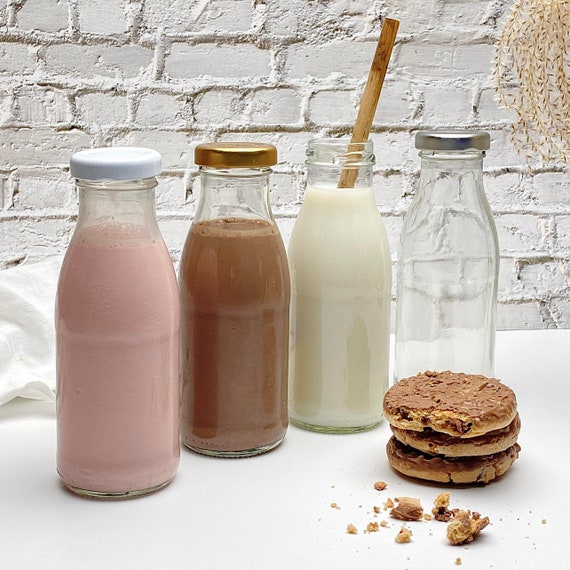The image showcases a minimalist setting with a white painted brick wall as the backdrop, adorned in the top right corner by what appears to be light brown branches or leaves. In the foreground, a white table holds four glass bottles arranged from left to right. The first bottle, capped with white, contains a pink liquid, likely strawberry milk. The second bottle features a gold cap and is filled with a brown liquid, presumably chocolate milk. The third bottle, uncovered and instead holding a wooden stir stick, contains white milk. The final bottle, sealed with a silver cap, is empty. Spread before these bottles is a small stack of three light brown cookies, likely chocolate chip, accompanied by scattered crumbs. Additionally, a white napkin can be seen behind the bottles, adding a subtle touch to the composition.